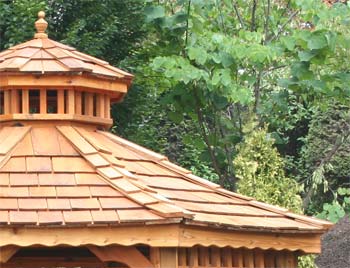The image is a color photograph taken outdoors, showcasing a picturesque wooden pavilion or gazebo with an elaborate, multi-tiered roof. This structure, possibly inspired by Asian architecture, is situated against a lush backdrop of green trees and foliage, which create the appearance of a forest. The roof is constructed from light-colored, new wood with no signs of weathering.

The pavilion features two distinct layers. The uppermost layer is crowned with a small decorative ball or finial, supported by small wooden beams. This layer is adorned with wooden shingles. Below it, the second section slopes outwards, also covered with wooden shingles, and is encircled by a scalloped edge that accentuates the intricate craftsmanship of the pavilion. The ornate carvings and architectural elements give the structure a distinctive, almost sacred feel, reminiscent of traditional Asian temples. The overall scene is serene, with the artfully constructed pavilion framed by the verdant greenery around it.